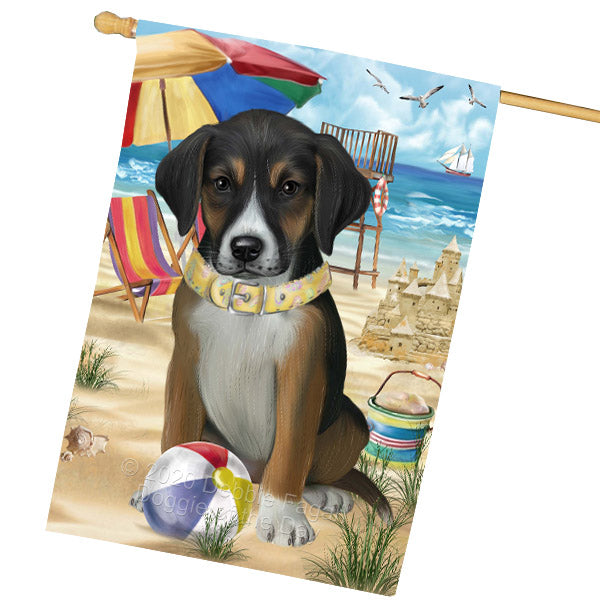This detailed description is for an image of an outdoor yard flag, affixed to a pole on the side of a home, depicting a charming beach scene. At the forefront, a brown Labrador with dark ears and a white chest sits contentedly with its paws forward, looking directly ahead. The dog's face features a mix of white, brown, and black, creating a pleasing contrast. Seated in front of a small, colorful beach ball, the dog is surrounded by playful elements: a multi-hued beach umbrella to its left, a vibrant beach chair, and a sand bucket right behind. The beach setting behind the dog includes a meticulously crafted, three-tiered sandcastle, a lifeguard chair, seagrass, and a serene ocean horizon with a sailing ship. Above, three seagulls soar against a cloudy sky. The scene is completed with the discreet text at the bottom of the flag, "2020 Debbie Fagan, Doggie of the Day." This idyllic beach tableau captures the joyful essence of a day at the beach with man's best friend.